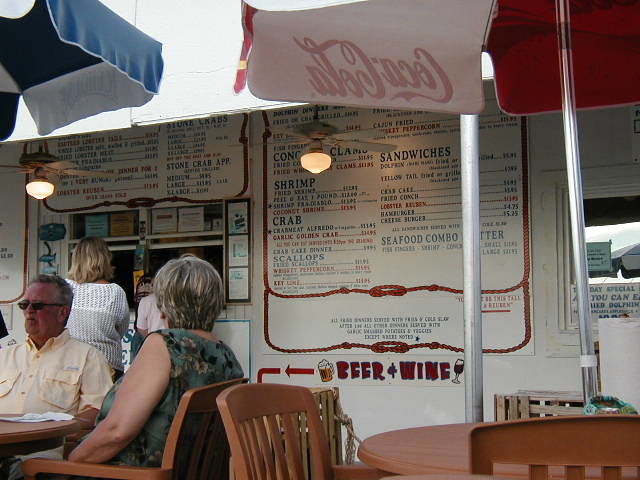This image depicts a lively outdoor setting at a restaurant known for its beer and wings. Central to the image is a small ordering window, at which a middle-aged woman is placing her order. In the foreground, an older couple is seated at a table beneath an umbrella, enjoying the ambiance. The man, distinguished by his small sunglasses and pale yellow shirt, has a notably flushed face, while the woman, dressed in a sleeveless green sundress, sports a short, dark brown hairstyle flecked with gray. Her upper arms are significantly paler than her sun-kissed lower arms. Also captured in the scene is an empty table to the right, waiting for new patrons. On the building around the window, various colorful menus have been painted, detailing the restaurant's offerings, which include sandwiches, shrimp, crabs, beer, and wings, though the specific dishes are not legible from the image. Overhead, two outdoor ceiling fans provide some respite from the warm weather, enhancing the inviting atmosphere of this outdoor eatery.